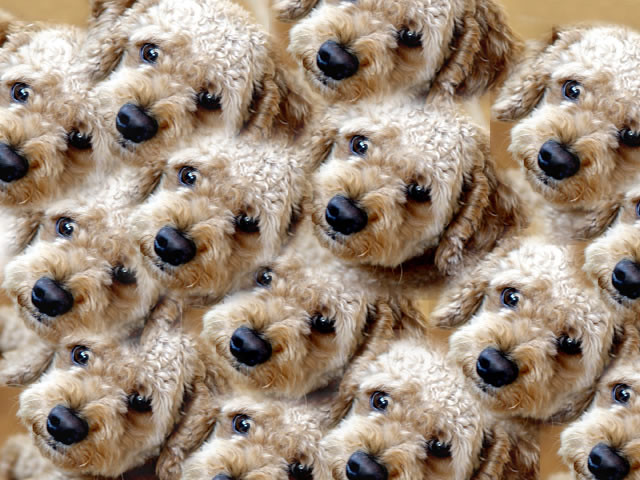The image features a computer-generated collage with a tan background, showcasing approximately 14 identical headshots of a fluffy, curly-haired puppy, likely a poodle or labradoodle with short, white fur. Each head has distinctly long, floppy ears, a black nose, and sad-looking brown eyes that gaze slightly to the left. The heads are tilted at a 45-degree angle and arranged diagonally from the bottom left to the top right, with some overlaps causing a slight blurriness at intersections. The pattern is irregular, creating a kaleidoscope-like effect rather than a perfect grid, and occasional glimpses of the light brown background peek through the gaps.